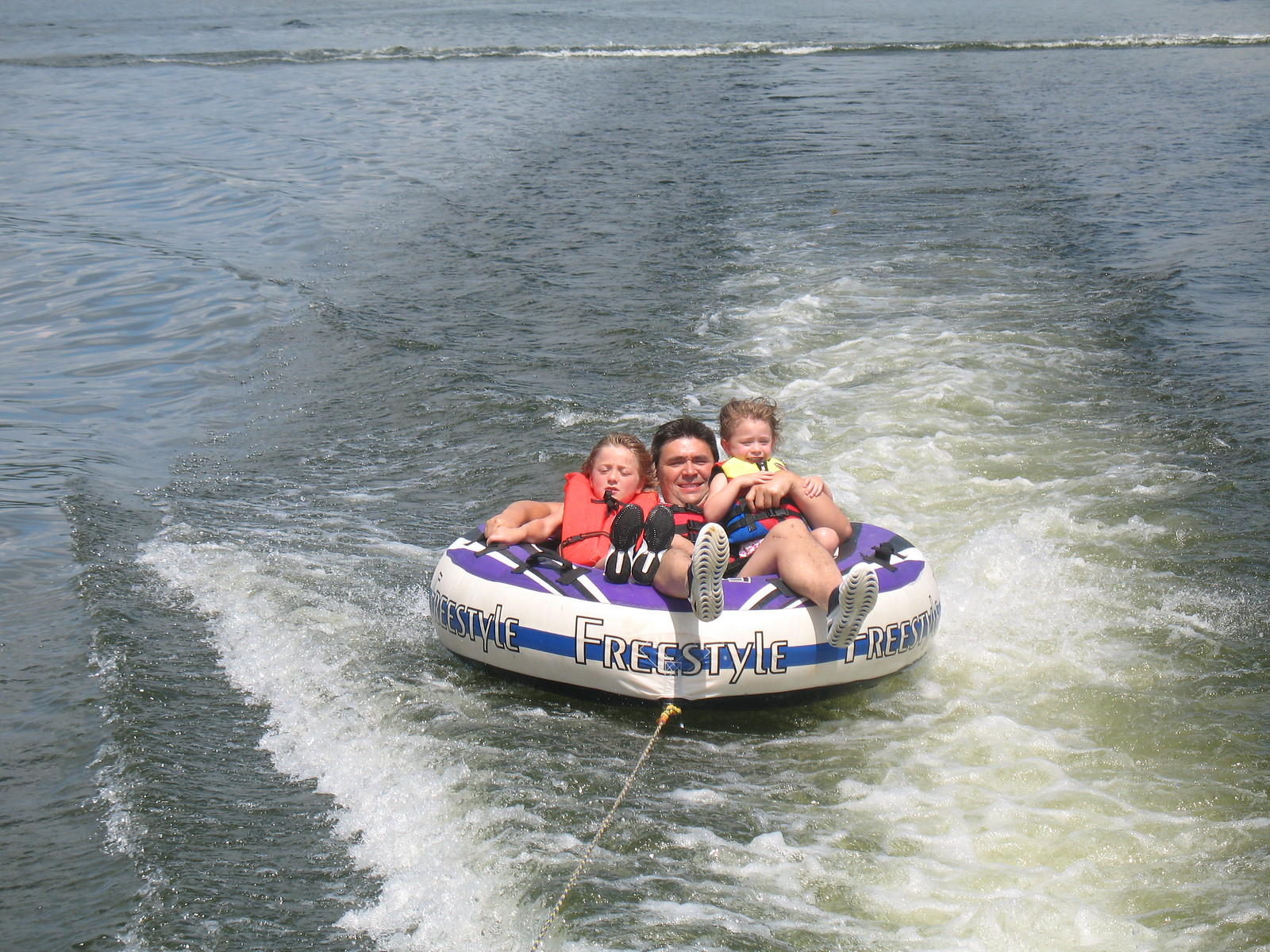In this colorful photograph, a grown man and two children are enjoying a thrilling ride on a purple, white, and black donut-shaped inner tube, emblazoned with the word "Freestyle" on a blue banner around its rim. The trio is being towed behind a boat by a brown rope, creating white ripples and a frothy wake in the blue water of a calm lake. Positioned in the center of the inner tube, the man, presumably the father, is flanked by a boy around eight years old on his left and a girl about four years old on his right. All three are secured in bright orange life vests, adding a layer of safety to their adventure. The father is wearing boat shoes with white soles, while the boy has boat shoes with black soles. The clear, serene water contrasts with the vibrant colors of the inner tube and their life vests, capturing a perfect moment of family fun and excitement on the lake.